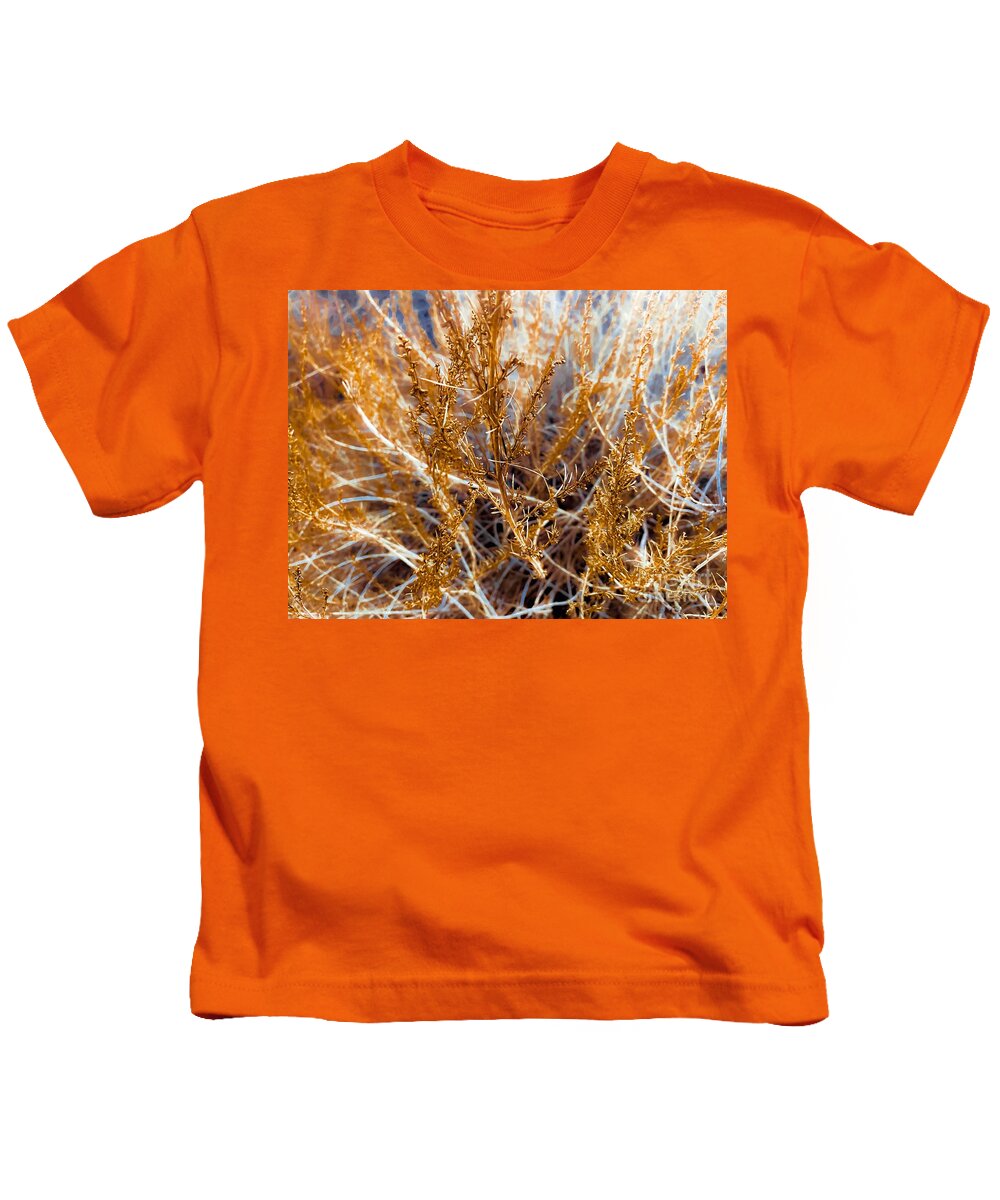A child's short-sleeved orange t-shirt is displayed against a white background. Centrally positioned near the collar of the t-shirt is an intricate graphic depicting an assortment of twigs, both brown and white, artistically arranged to resemble a bush. The vibrant orange fabric contrasts sharply with the white backdrop, drawing attention to the detailed twig design.